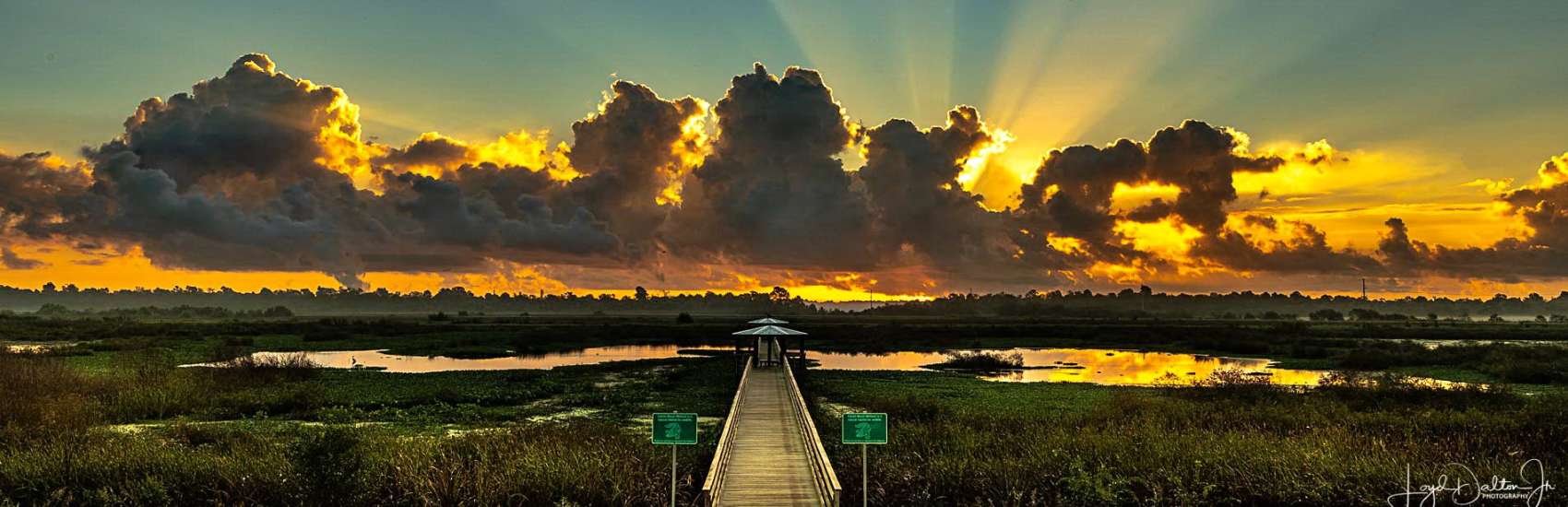The photograph captures a picturesque, sunset scenery featuring a wooden dock that stretches out towards a tranquil body of water, possibly a lake or a small bay. The dock, equipped with two umbrellas at its end and park-like green and white signs along its sides, offers a picturesque spot for relaxation by the water. Above, the sky is a dramatic tapestry of dark grey and white puffy clouds, with the sun setting behind them, casting a captivating mix of light and dark hues across the landscape. The sunlight breaks through the clouds, casting orange rays that illuminate the water and the backdrop of distant mountains. The lower right corner of the photograph is signed by Lloyd Dalton, adding a personal touch to this serene and visually stunning scene.